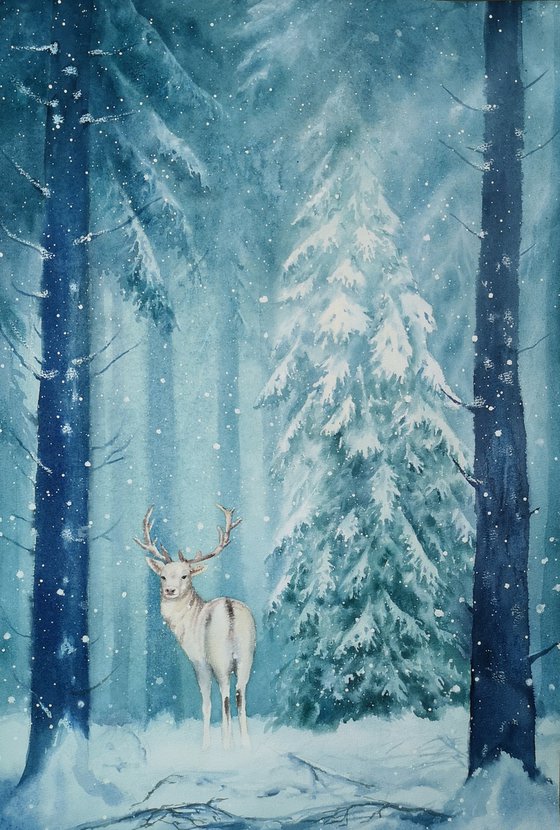This detailed piece of art depicts a serene winter scene, featuring an albino deer standing in a snow-covered forest. The deer, with striking white fur and antlers, has dark eyes that gaze back toward the viewer, giving a sense of cautious curiosity. The foreground showcases two large, gray trees with sparse branches and several fallen branches scattered on the snowy ground, suggesting they may have recently fallen. The background is a beautiful array of tall evergreen trees and various tree trunks, some heavily laden with snow that appears freshly dusted, akin to a powdered sugar coating. Snowflakes are gently falling, adding to the scene's tranquil ambiance. The composition, reminiscent of a magical winter wonderland straight out of Narnia, captures the deer's moment of pause before it seemingly turns to disappear back into the dense, snow-laden forest. The illustration is tinged with subtle blue hues, enhancing the cold, serene atmosphere of this enchanting winter scene.